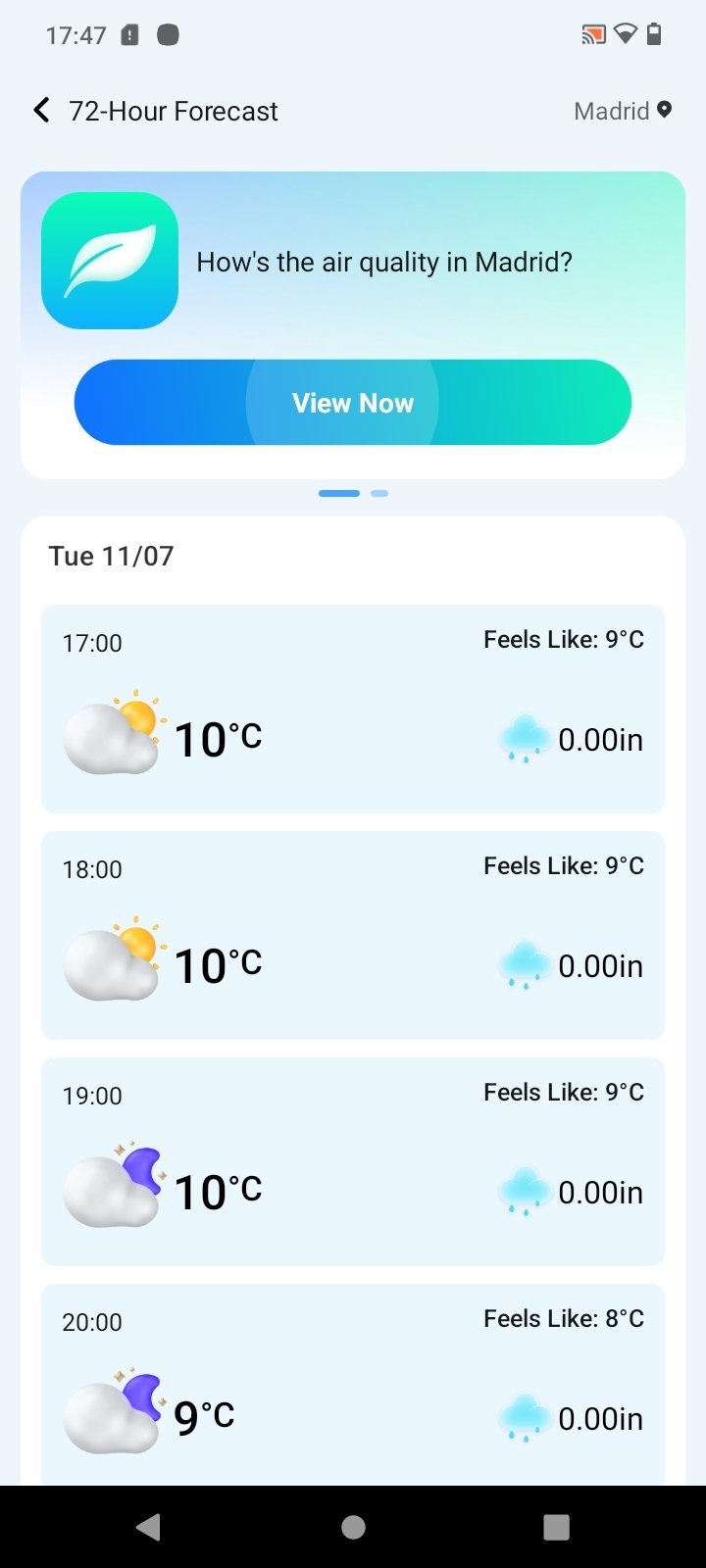The image features a light blue background with a variety of informational elements related to weather and air quality. 

At the top, the screen displays the device's time, 17:47, located near Wi-Fi and half battery signal icons. Centrally placed, the text reads "72 Hour Forecast in Madrid." 

Beneath this headline, a turquoise-colored box with a white leaf graphic indicates "Air Quality in Madrid." A blue button labeled "View Now" is positioned below this box.

Further down, detailed hourly weather information for Tuesday is presented:
- At 11:07, the temperature is 10°C, which feels like 9°C.
- At 17:00, the temperature remains 10°C, feeling like 9°C.
- At 18:00, it again reads 10°C, with a perceived temperature of 9°C.
- At 19:00, the temperature stays at 10°C, still feeling like 9°C, with no precipitation recorded (0.00 inches).
- Finally, at 20:00, the temperature drops to 9°C, feeling like 8°C, with no precipitation detected (0.00 inches).